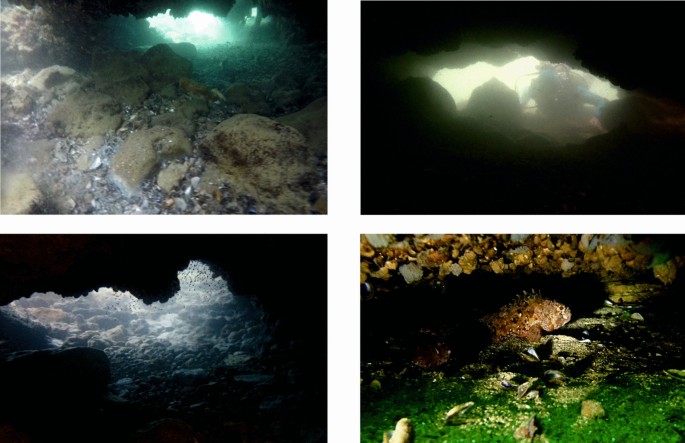These are four underwater images, likely taken while scuba diving, showcasing various sections of an underwater cave system. 

In the upper left image, a jagged, rocky area is visible, illuminated by a light source filtering through the cave's entrance. The scene, predominantly brown and tan with some visible debris and seashells in the crevices, extends into a darker tunnel with a bluish light tinting the distant background.

The upper right image captures a dimly lit scene with a pale rock formation at the center. A scuba diver, partially visible in a blue jumpsuit and carrying equipment such as an oxygen tank, is faintly outlined against the darkness.

The bottom left image portrays a deep section of the cave, where the black, rocky surroundings give way to a lighter area in the center. The uneven surface here is strewn with pebbles and stones, and the light appears to be coming from above.

Finally, the bottom right image shows a dimly lit underwater scene with a bit of green algae visible at the front. Among the rocks, a brown, bumpy-textured fish with fins along its back is noticeable, looking towards the right side of the image. The overall illumination is minimal, hinting at the isolation of this cave section.